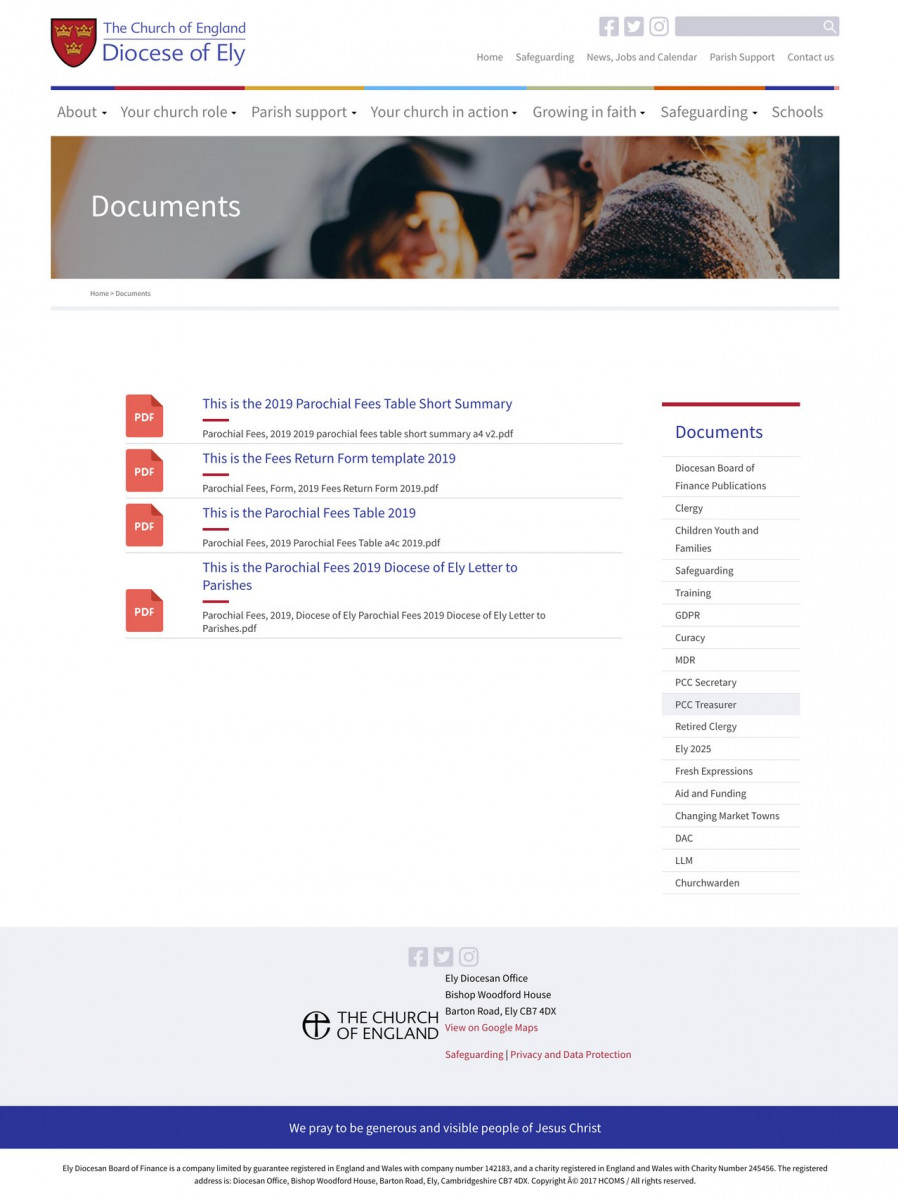A screenshot from the Church of England, specifically the Diocese of Ely. The image features a white background with notable elements including:

- **Top Left:** A red shield adorned with three gold crowns, signifying the emblem of the Diocese of Ely. Below the shield, in grey text, the words "The Church of England" are displayed. Directly underneath, in prominent, bold text, is "Diocese of Ely."
- **Top Right:** Icons for Facebook, Google, Twitter, and Instagram are positioned alongside a search bar.
- **Below the Upper Elements:** A navigation menu lists the following options - Home, Safeguarding, News, Jobs and Calendar, Parish Support, and Contact Us. A colorful line with blues, yellows, reds, and greens runs beneath this menu.
- **Secondary Navigation:** In grey text, additional categories are outlined - About, Your Church Role, Parish Support, Your Church in Action, Growing in Faith, Safeguarding, and Schools.
- **Main Image:** A photograph capturing a group of white individuals standing together, laughing. To the left of the image, a white text box labeled "Documents."
- **Document Section:** Four red icons with "PDF" in white font listed vertically. These documents include titles like "2019 Parish Fees Table," "Fees Returned for 2019," "Parish Fees Table 2019," and "Parish Fees, Diocese of Ely, Letter to Parishioners."
- **Right Sidebar:** Additional information about various documents and resources available.
- **Bottom Bar:** A purplish-blue bar extending across the bottom of the page.

This detailed description captures the essence and layout of the Church of England, Diocese of Ely's webpage as shown in the screenshot.